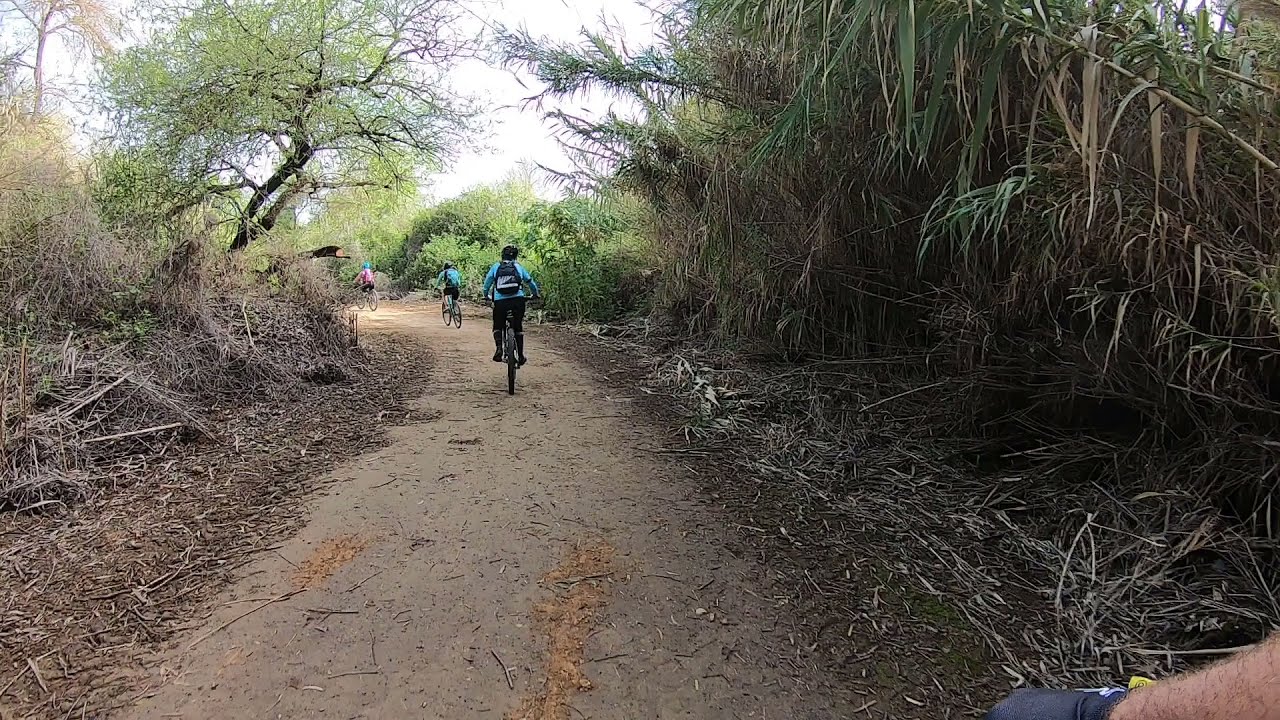This color, landscape-oriented image appears to be a still from a GoPro camera mounted on the helmet of a cyclist riding on a winding dirt trail through a forested area. The trail, starting prominently in the foreground, curves and recedes into the background, eventually vanishing from sight. Three cyclists are ahead on the path, moving deeper into the forest. The closest cyclist, distinguished by a light blue top, black helmet, pants, socks, shoes, and a backpack, is followed by a second cyclist in a light blue top, black shorts, and a black helmet. The furthest cyclist is donning a pink top, blue helmet, and black shorts. The trail is flanked by trees, bushes, fallen branches, and both dead and green foliage. To the right of the riders, there is a significant bamboo grove, while the left side is characterized by more trees and dead grass. The background reveals a bright, sunny sky with hazy lighting filtering through the distant trees, indicating a daytime setting. All cyclists are wearing helmets, immersed in their journey along this picturesque forest trail.